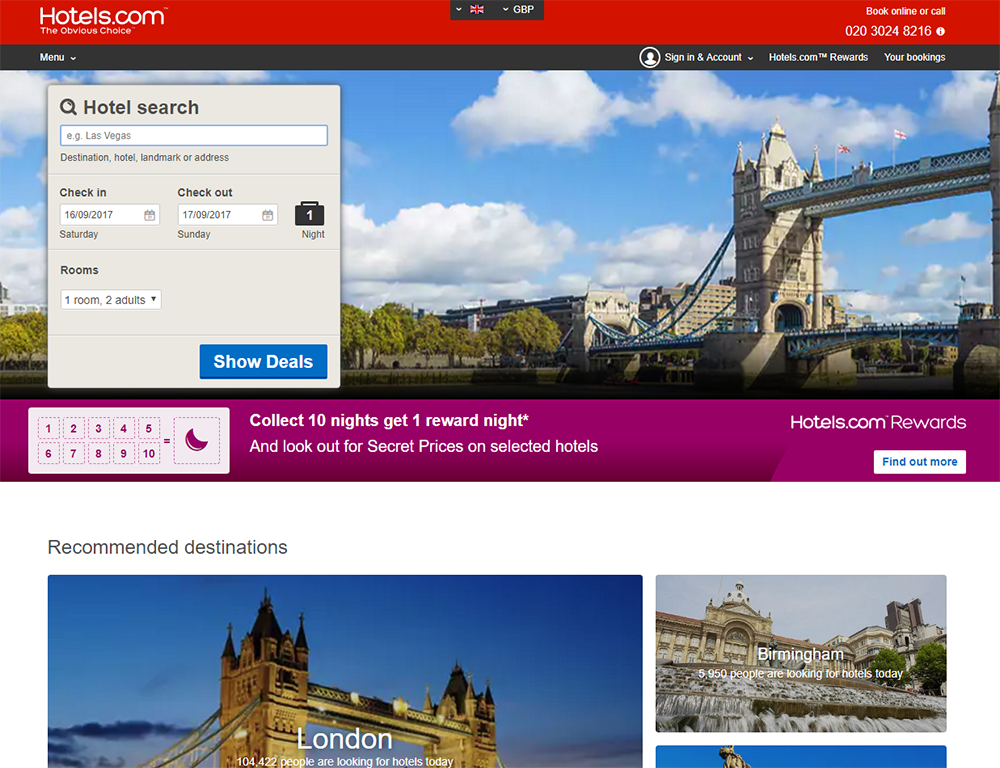Screenshot of the Hotels.com Homepage: 
The image depicts the homepage of Hotels.com, prominently featuring the company's logo in red at the top. A menu button is visible, allowing users to initiate a hotel search. The search box provides examples of potential queries, such as a destination, hotel, landmark, or address. 

A navigation bar is present, offering options like "Back Online or Call," accompanied by a support phone number for assistance. Users have the ability to sign into their account, access the rewards section, or check their bookings. This feature is particularly useful for travelers who need to keep track of their reservations, like those planning an extended stay in London.

The central hotel search section includes a dialog box for entering a desired city. Users can enter check-in and check-out dates manually or by selecting dates from an interactive calendar, which updates the number of nights accordingly. There is also a drop-down menu to choose the number of rooms and guests, with options such as one room for two adults or two rooms for four adults.

At the bottom of the image, a promotional message highlights the Hotels.com rewards program: "Collect 10 nights, get 1 free," and entices users to look out for secret prices on selected hotels. This comprehensive homepage allows users to sign in, search for accommodations, or enjoy member benefits seamlessly.